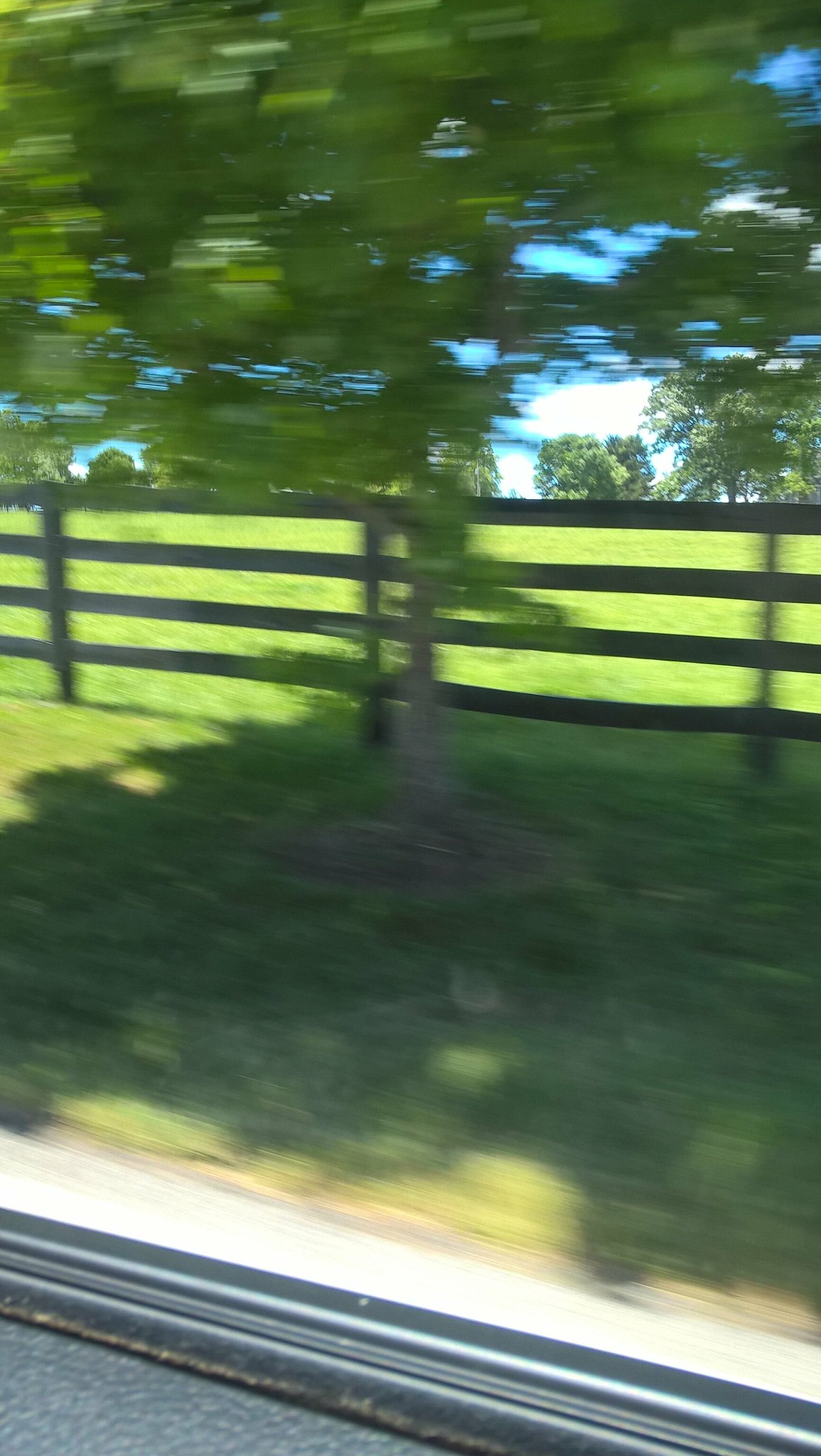The photo captures a fleeting moment from the side window of a moving car, resulting in a slightly blurry image. The bottom portion of the picture reveals the slanted car window frame, extending from the bottom left-hand corner toward the upper right-hand side. Outside, a landscape of vibrant nature unfolds, dominated by lush trees that frame a clear blue sky adorned with patches of fluffy white clouds. Beneath the trees, a wooden fence stretches horizontally, providing a rustic touch. Just in front of the fence and next to a tree, a small, indistinguishable animal adds a sense of mystery due to its blurriness. Sunlight filters through from above, casting shadows on the ground from the left-hand side, leaving patches of bright green grass illuminated next to the car. Beyond the wooden fence lies a field of even greener, lighter-shaded grass, enhancing the idyllic scenery.